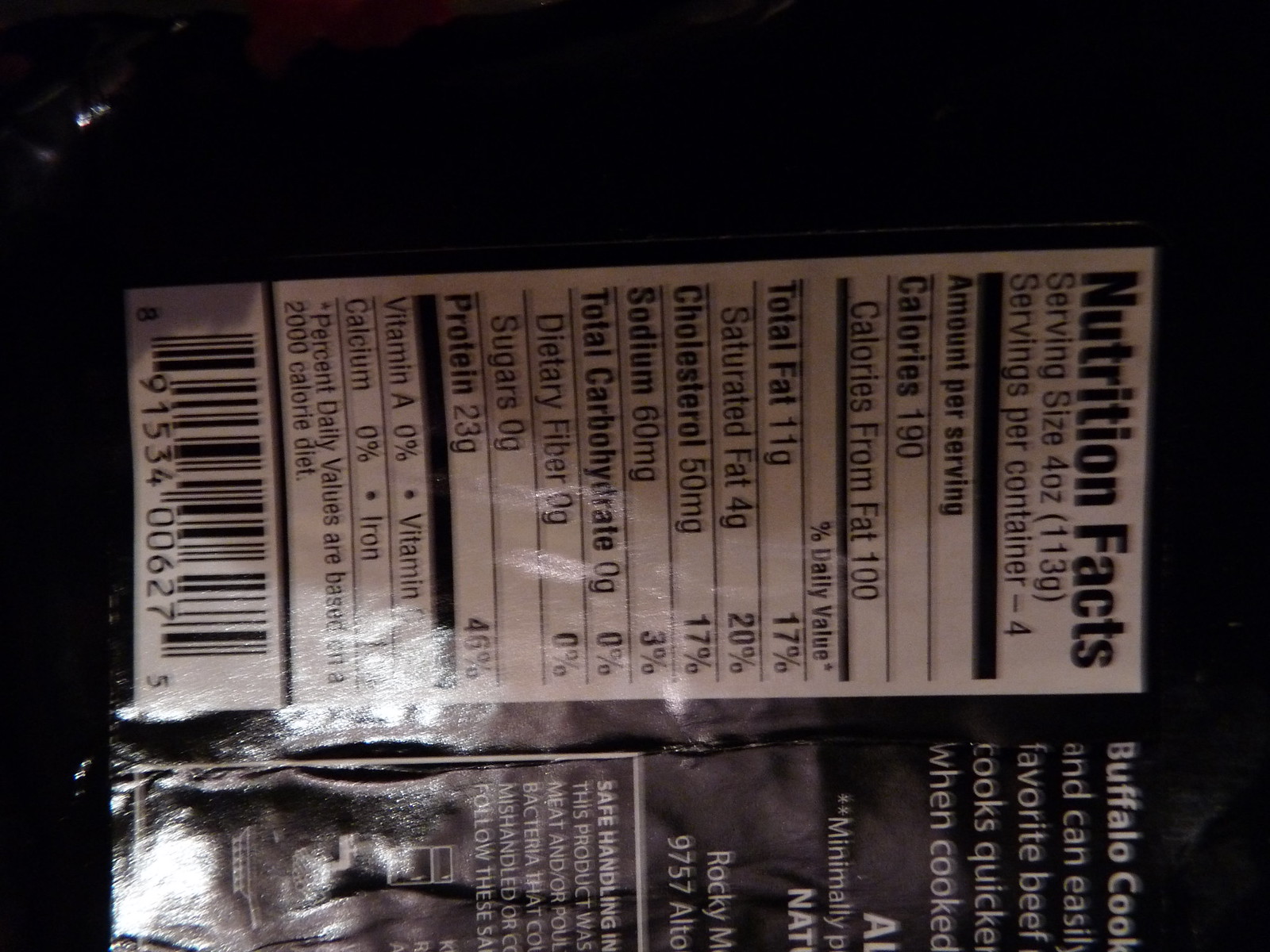The image shows a photograph of a food package label, positioned sideways against a completely black background. The label has white text on a brown background and prominently displays the nutrition facts. The label reads:

"Nutrition Facts: Serving size 4 ounces (113 grams). Servings per container: 4. Amount per serving: Calories 190, Calories from fat 100, Total fat 11 grams (17% DV), Saturated fat 4 grams (20% DV), Cholesterol 50 milligrams (17% DV), Sodium 60 milligrams (3% DV), Total carbohydrate 0 grams (0% DV), Dietary fiber 0 grams (0% DV), Sugars 0 grams, Protein 23 grams (46% DV), Vitamin A 0%, Calcium 0%."

The bottom of the label has a barcode (UPC code) with numbers beneath it. There is partially legible text which includes, "buffalo cook and can easily favorite beef, cooks quicker when cooked," and some other cut-off words. The label suggests the product is some type of meat, likely buffalo, with minimal processing.